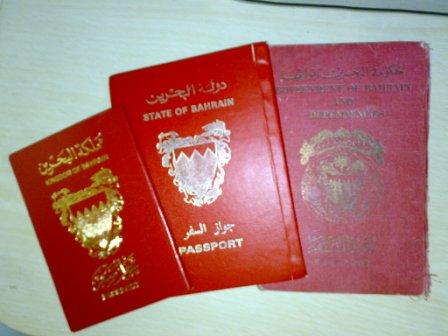On a wooden surface, three red passports are carefully arranged, each bearing the State of Bahrain's emblem in various states of wear and clarity. The central passport prominently displays "State of Bahrain Passport" in gold text with a shimmering gold crest, further highlighted by what appears to be camera flash, making it the most distinguishable. The other two passports, although not entirely legible, also seem to belong to the State of Bahrain, featuring similar gold writing and crests. The passport on the left appears to be smaller, with a prominent gold crest, while the one on the right is notably faded, showing signs of age and a tear in the bottom right corner. The text on these passports includes both English and Arabic script.